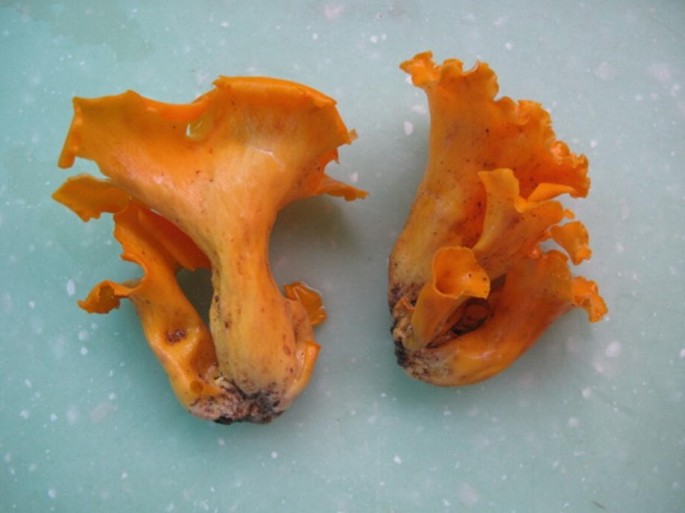The image captures a top-down view of two clusters of mushrooms set against what appears to be a robin's egg blue countertop with white speckles, resembling a granite finish. Each orange mushroom displays a fluted, ruffled texture and tapers outwards from their bulbous bases, which are flecked with black and brown dirt. The left cluster features one prominent mushroom at its center, flanked by a smaller mushroom on its left and a very tiny one on its right. Similarly, the right cluster boasts four mushrooms of varying sizes: a large one at the back, two medium-sized ones in front, and a smaller one at the forefront. The mushrooms exhibit a spectrum of orange hues, ranging from pale yellowish tones to vibrant, bright oranges, with some streaks of lighter orange interspersed throughout.